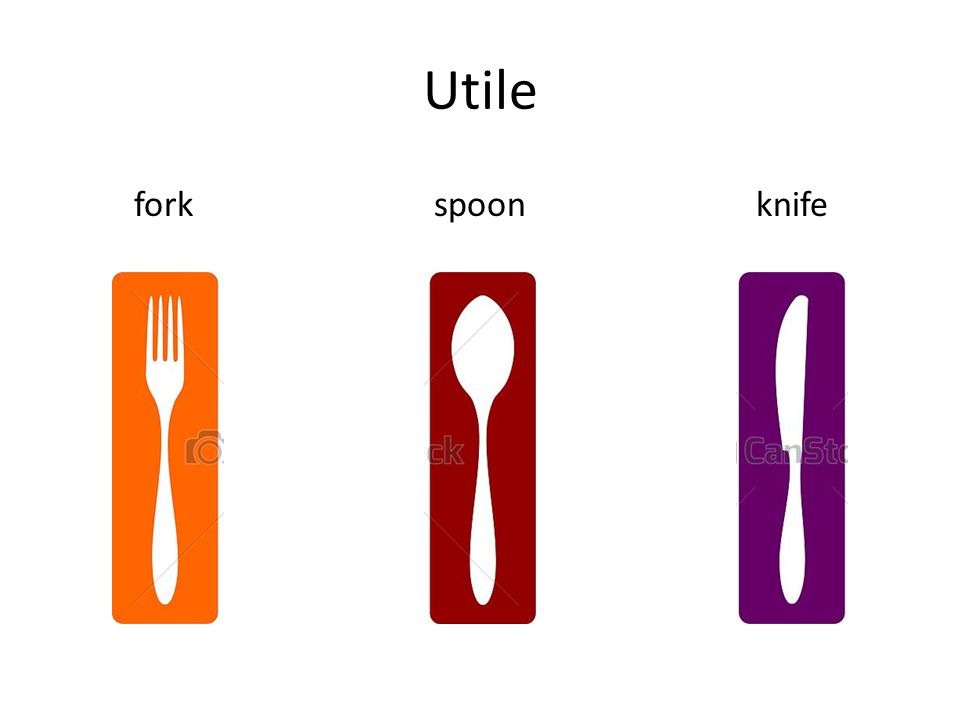The image is a diagram or illustration on a white background featuring three vertical rectangles, each showcasing a different utensil. At the top, in black letters, it reads "Utile." On the left is an orange rectangle with a white fork, and above it, the word "Fork" is written in black. In the middle, a maroon rectangle contains a white spoon, with the word "Spoon" in black above it. On the right, a purple rectangle depicts a white butter knife, and above it, the word "Knife" is written in black. The entire image appears to be styled as an informative graphic, perhaps for a menu or a website, with an unreadable light watermark over the spoon and knife.